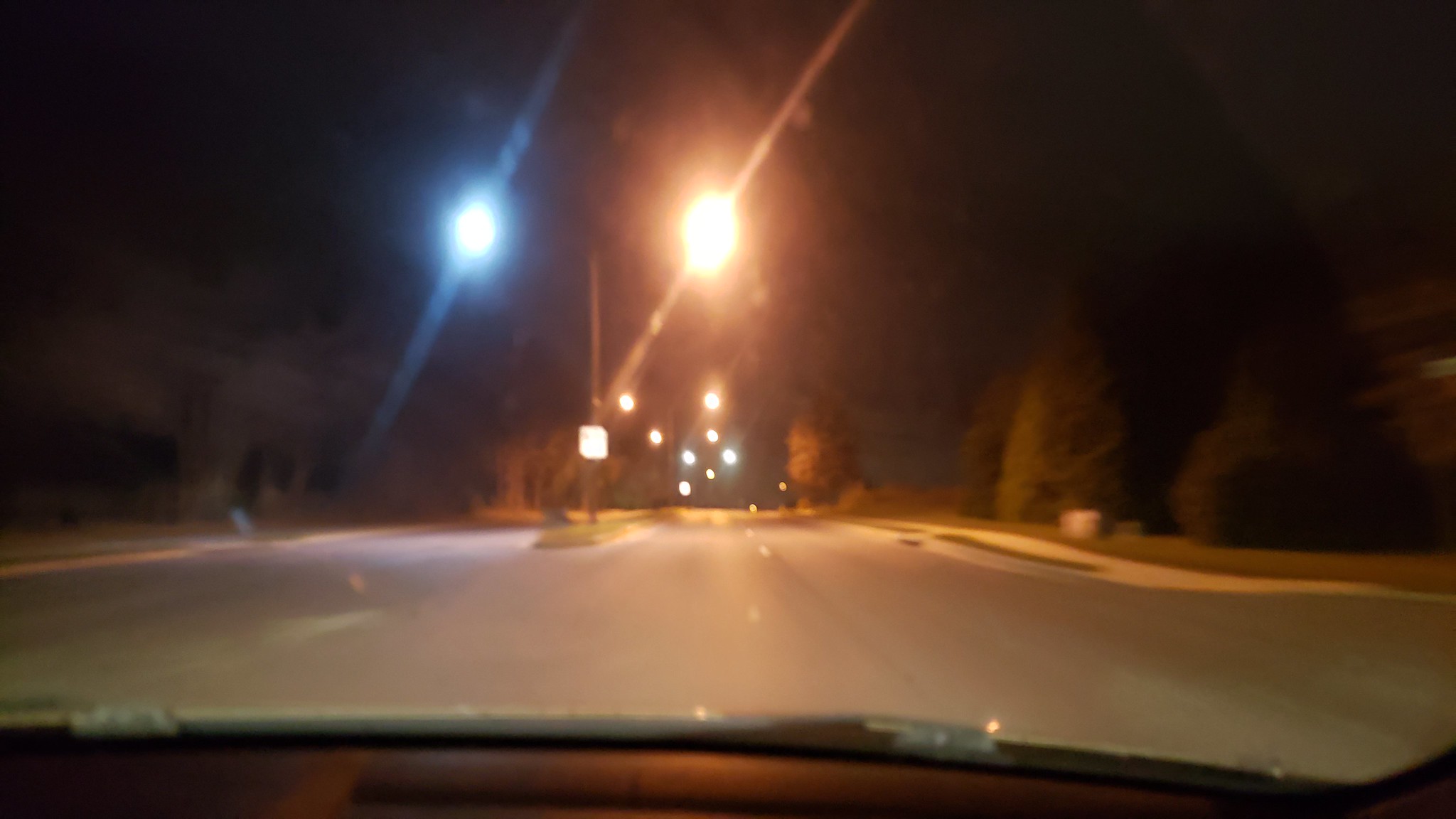A nighttime street scene viewed from inside a vehicle showcases a clear black concrete road. The camera angle reveals a distant dark sky punctuated by two vividly bright lights. One light radiates a blue hue while the other emits an orangey-reddish glow, their reflections creating striking patterns across the sky. Flanking the street are lush green trees, including one shaped like a classic Christmas tree, dense with foliage. On the left side of the image, a building is partially visible, adding an urban element to the serene night setting.